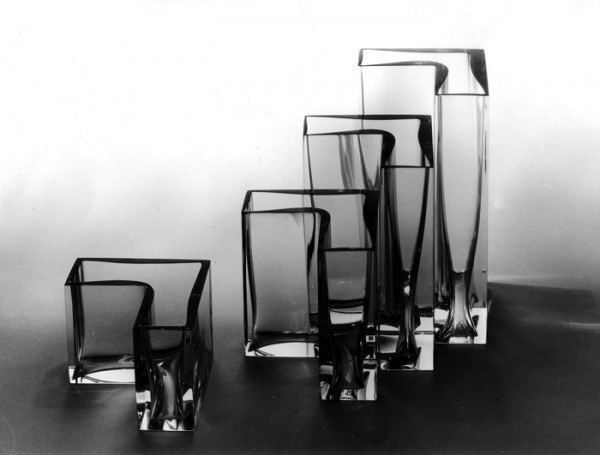This image showcases a series of four transparent L-shaped glass containers, arranged in ascending order from left to right. The containers, appearing empty and pristinely clean, are incrementally taller as you move rightward, with the shortest being on the far left and the tallest on the far right. The containers nestle closely together, fitting neatly into one another, and they are centrally positioned within the square frame of the photo.

The backgrounds and surface create a gradient of colors: starting from a bright white at the top, transitioning through a medium gray in the middle, and ending in a charcoal to black shade at the bottom. This gradient backdrop highlights the clear, transparent nature of the containers. The image is devoid of any text or additional objects, presenting a minimalist and organized setting that suggests an indoor environment, perhaps a kitchen table or counter.